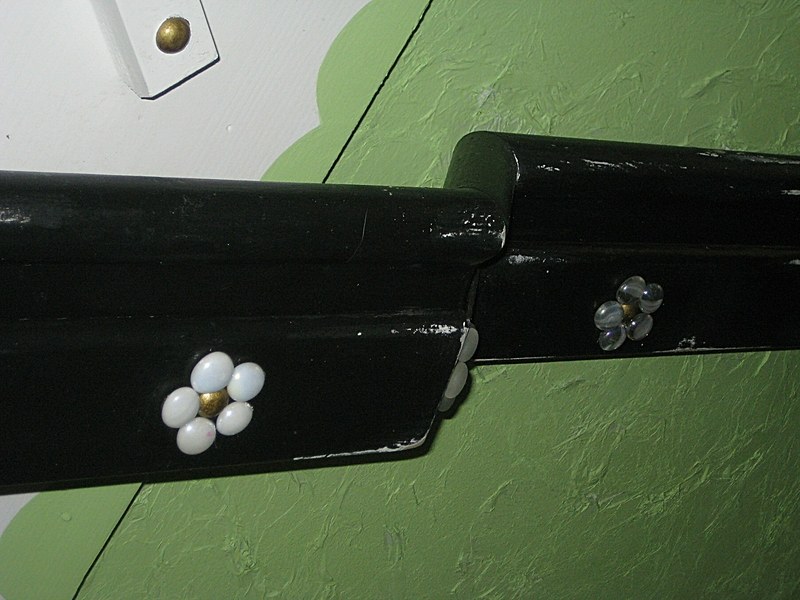The image features three purses placed on a green surface, likely a table. Two of the purses are black and shiny, adorned with decorative white flowers that have gold centers. Behind them, there is a white purse with a gold button enclosure. Alongside these items, there are black wood trim pieces with decorative beads attached, which do not align perfectly, creating a mismatch in the border where they meet. The background of the image includes both a green textured surface and a smoother green wall area with a noticeable transition to a white section on the left.